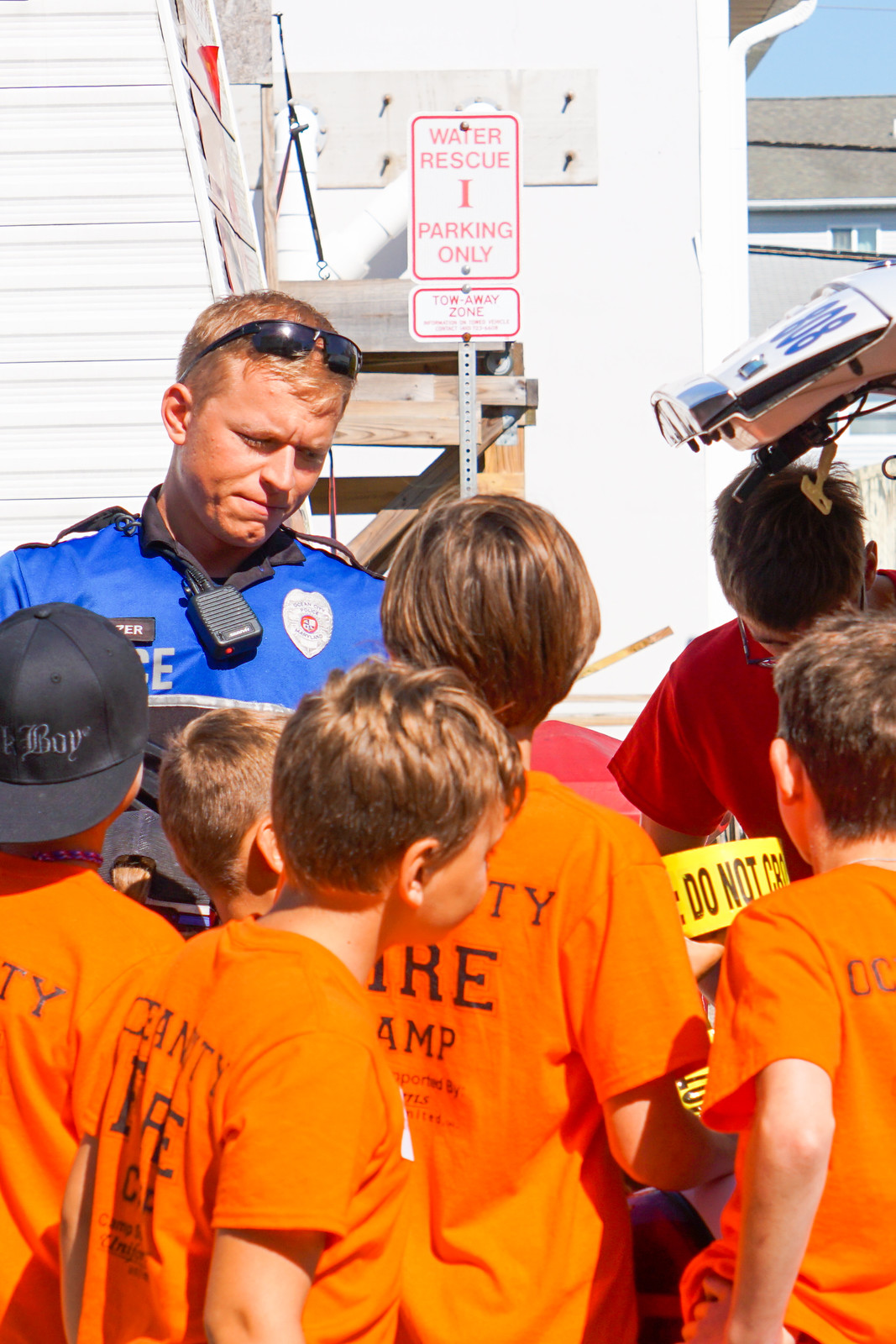In this outdoor photograph, a group of children dressed in bright orange t-shirts with black print, which appears to say "County Fire Camp," are facing away from the camera. They seem to be engaging with a police officer who stands in front of them, slightly to the left. The officer, wearing a blue shirt with the word "police" printed in white and a silver badge on the lapel, has black sunglasses perched on his head and a radio or microphone around his neck. The officer seems attentively listening to one of the boys who is holding on to yellow "Do Not Cross" police tape. This scene appears to be taking place near a beach or by a body of water, as indicated by a sign in the background that reads "Water Rescue Parking Only," bordered in red against a white background. Additionally, there's a camera apparatus visible in the upper right part of the image pointing towards the officer, adding to the detailed setting of this engaging moment.